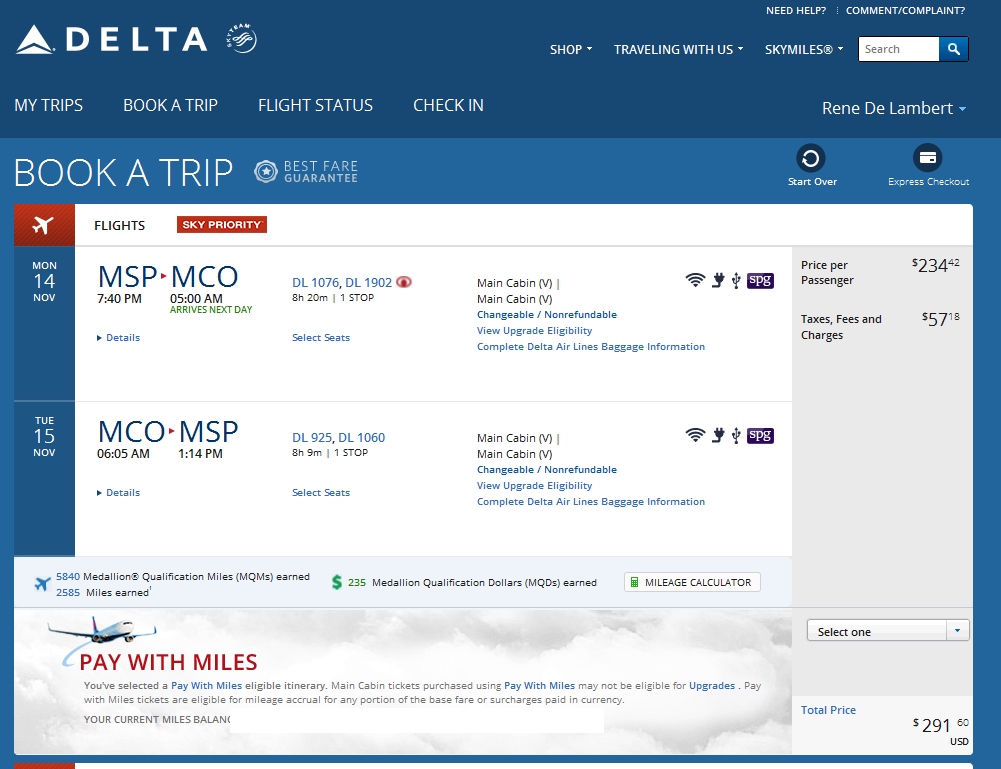**Caption:**

A screenshot from the Delta Airlines website, displayed in a square, 4:3 aspect ratio format often associated with older devices or tablets. The interface exhibits a modern design with a dominantly blue color scheme and a blue border at the top. In the upper left corner, "Delta" is prominently displayed in white capital letters alongside the airline's logo, a stylized triangle with a line through it.

The navigation bar offers various clickable links such as "Shop," "Traveling with Us," "SkyMiles," and includes a search box with a magnifying glass icon. Below the navigation bar are clickable tabs for "My Trips," "Book a Trip," "Flight Status," and "Check-In."

The user, Rene de Lambert, is currently logged in. The main content area visible shows options for booking a trip, with an existing booking for Monday, November 14th, and Tuesday, November 15th. Although the destination is not legible due to the image quality, the total price for the flight is partially visible at $291 and some cents.